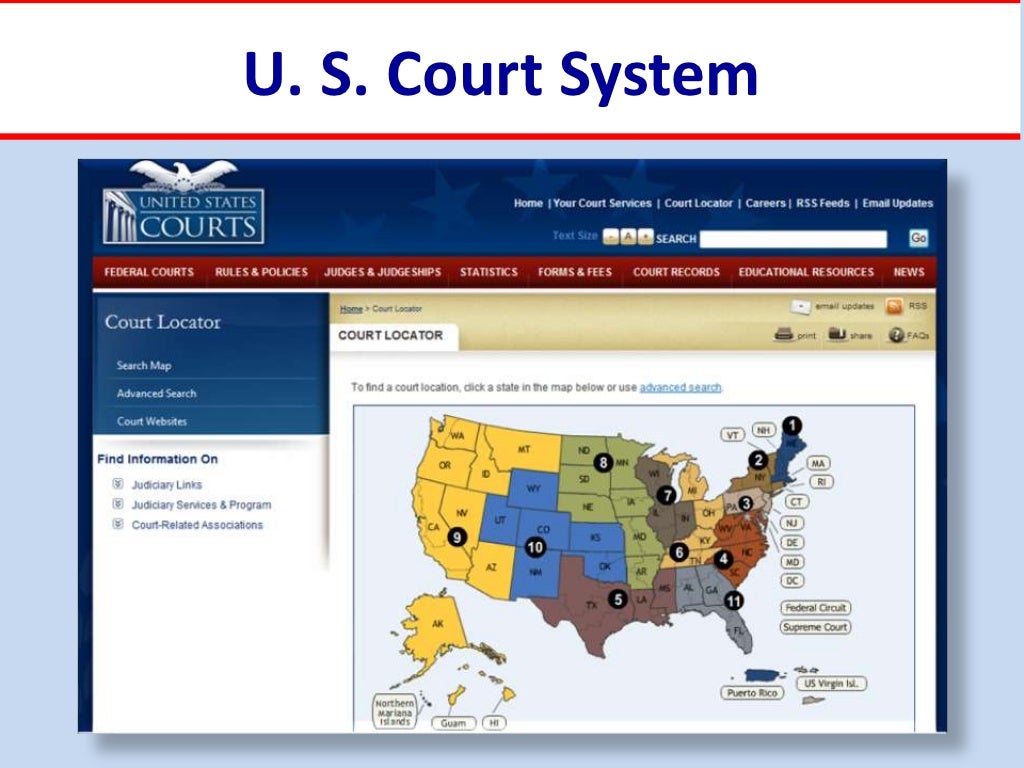The webpage belongs to the US Court System and features a prominent blue heading at the top. On the top left, there is a piece of artwork depicting a white eagle, beneath which the text "United States Court" is displayed. To the right of this, a series of navigation buttons are aligned horizontally, labeled as follows from left to right: Home, Your Court Services, Court Locator, Careers, RSS Feeds, and Email Updates. Below this navigation menu, a white search bar is positioned with the word "Search" on the left side and a "Go" button on the right side.

Further down the page, there is another row of tabs spanning from left to right, labeled as: Federal Courts, Rules and Policies, Courts and Judgeships, Statistics, Forms and Fees, Court Records, Educational Resources, and News. Lastly, on the left side of the subsequent section, a vertical list of tabs labeled Court Locator is visible, arranged from top to bottom.